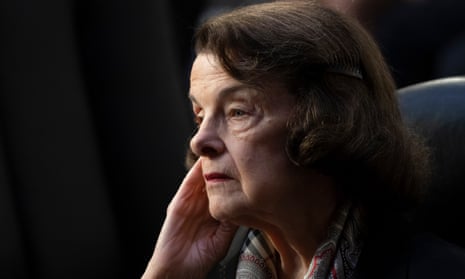This is a detailed portrait of Dianne Feinstein, an elderly white woman, likely taken before her death, when she appeared to be in her 70s. She is seated in a leather chair, positioned against a completely black background that lacks any discernible details. Dim lighting creates a dramatic contrast, with light sourced from the left casting heavy shadows on the right side of her face. Feinstein's face, framed by mostly dark brown hair interspersed with streaks of gray, displays a pensive and somewhat suspicious expression as she gazes off to the left. Her right hand rests thoughtfully against her cheek, accentuating her contemplative demeanor. The photograph captures her from the shoulders up, rendering her attire indistinct, though she appears to be wearing a striped shirt. The overall lighting and composition of the image highlight the textures of her hair and the reflection on the leather chair.